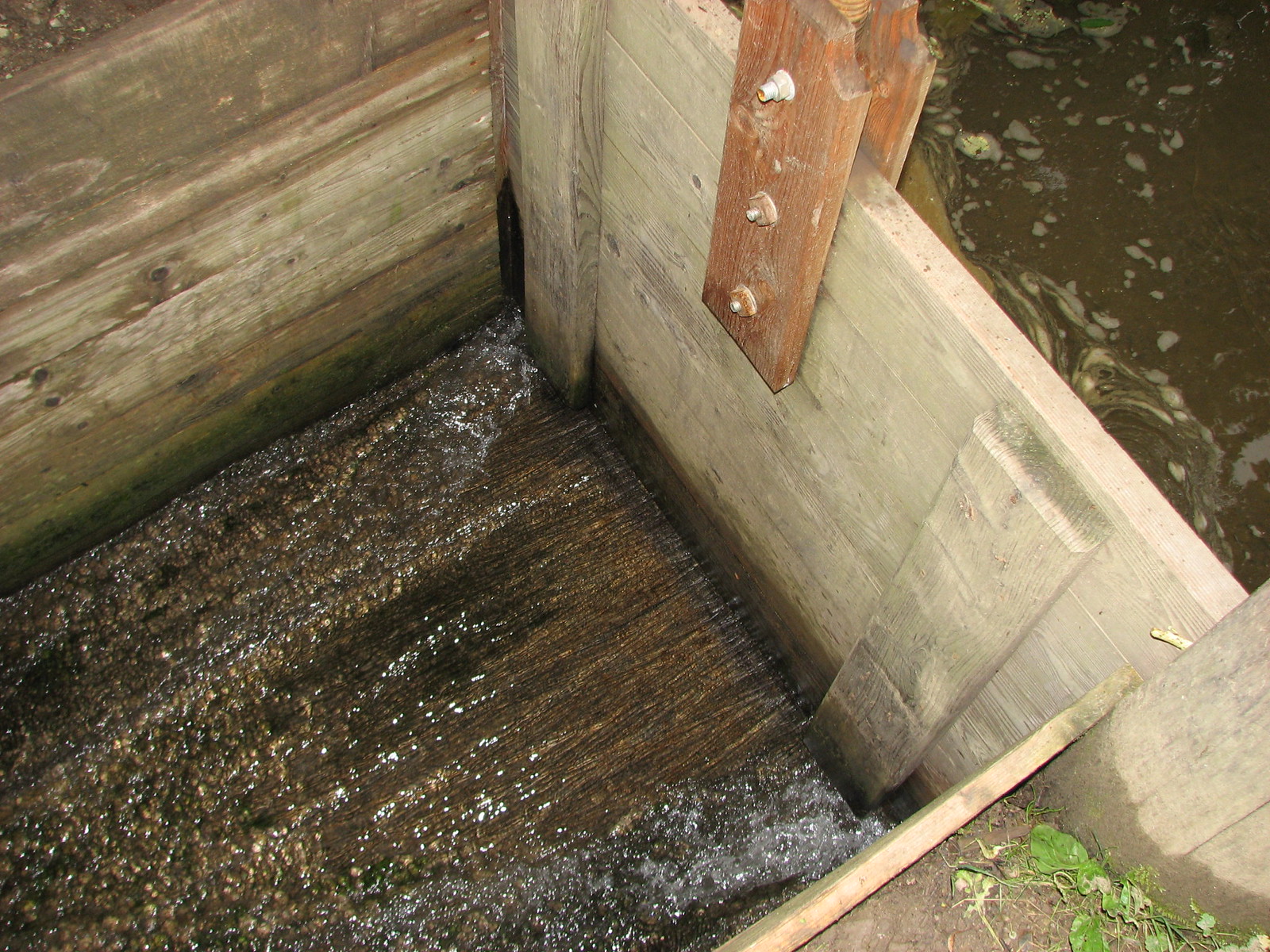The image showcases a wide rectangular wooden structure that resembles a sluice gate or an irrigation canal. The interior walls and floor are made of dark brown wooden panels, which appear to be covered with a shiny substance or possibly ice. The wooden panels form a well-defined enclosure, with the structure extending diagonally from the bottom right corner to the upper left, creating a sense of depth in the photo. On the top short side of this enclosure, there's an orange wooden component with three screws ascending vertically. In the bottom right corner, amidst what appears to be waterlogged patches, there is some dirt with green leaves. The water in the canal looks murky and unappealing, filled with green and brown sludge, indicative of its stagnant nature. At the far end, a door with a handle at the top center suggests a mechanism for controlling water flow, likely sliding up to allow water from an adjacent body of water, perhaps a pool or river, to flood the canal for irrigation purposes.